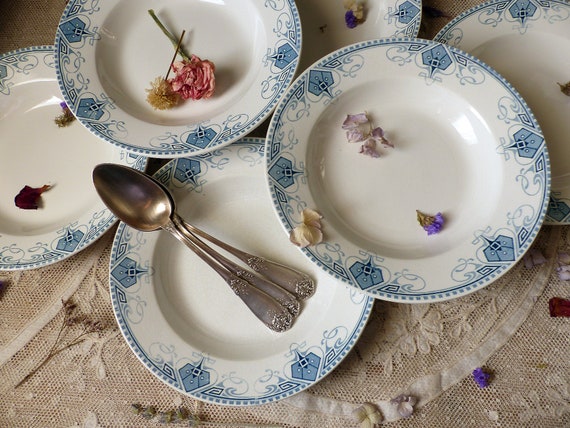In this image, a set of six round, fine china plates is elegantly arranged on a white linen tablecloth with a floral pattern. The plates are notably sophisticated, with a white interior bordered by a decorative blue pattern featuring triangular shapes divided into three sections, along with intricate twists and dotted trim. Each plate has a slight recessed saucer bowl, enhancing their delicate appearance. The table is garnished with scattered flower petals and heads, adding a splash of vibrant color to the composition: a red flower on the top-left plate, and a mix of white, purple, and light purple petals on the front-right plate. Additionally, three silver spoons, displaying a floral inlay design on their handles, rest on the left side, further contributing to the vintage charm of the scene.